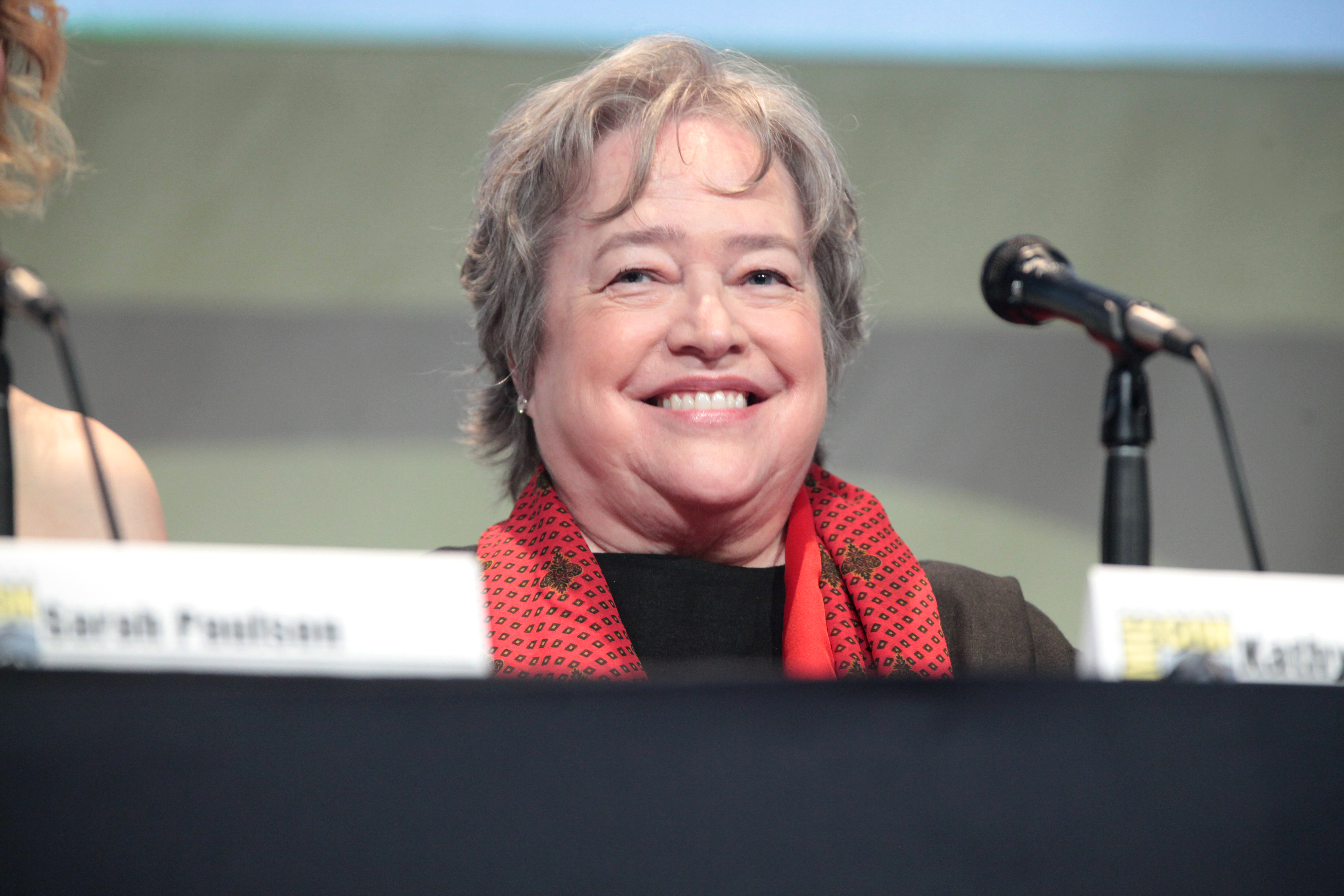In this photograph taken at Comic-Con, Kathy Bates is seated behind a black table, partially obscured by a white paper with the Comic-Con logo in yellow and part of her name visible, although blurry. She is positioned in front of a black microphone on a stand with a black cord. To her left, we can see the hair of another woman, also in front of a microphone, indicating a panel discussion. Bates is smiling warmly and looking slightly to her left. She is wearing a layered outfit consisting of a brown or dark gray jacket, a black shirt, and a red scarf with a rectangular, tilted square pattern, possibly silk. Her hair, a mix of graying shades, is short, slightly messy, and falls onto her forehead. The background behind her is out of focus, featuring mostly grays with a touch of blue, suggesting a stage setting. Despite some elements being blurry, the image captures Bates' engaging presence and the lively atmosphere of the event.